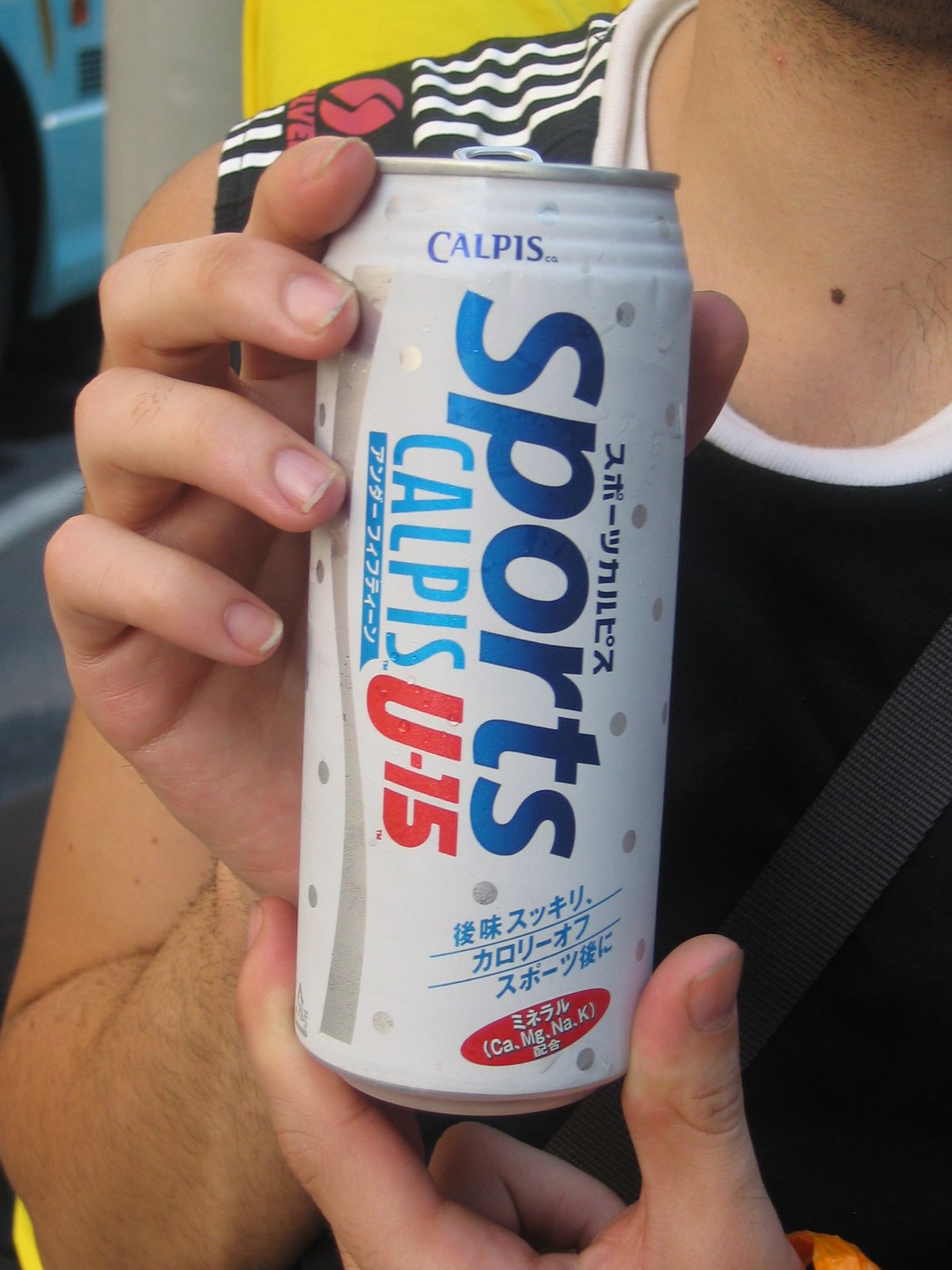In this color photograph, a partial view of a person, believed to be a woman with pale skin and delicate fingers, is depicted, revealing her neck and part of her torso. She is wearing a sleeveless black shirt with a scalloped neckline that features a white outline and white stripes on the shoulders. The focus of the image is the white, tall and slim tin can she is holding with both hands, which has dirty fingernails. The can features a silver vertical banner running from bottom to top. At the top of the can, "C-A-L-P-I-S" is vertically written in small blue letters, followed by the word "sports" in bold blue letters. Beneath this, "C-A-L-P-I-S" is written in light blue, and "U-15" in red letters. The lower portion of the can contains writing in what appears to be either Chinese or Japanese, adorned with silver dots scattered across the surface. In the background, hints of yellow and blue are visible.